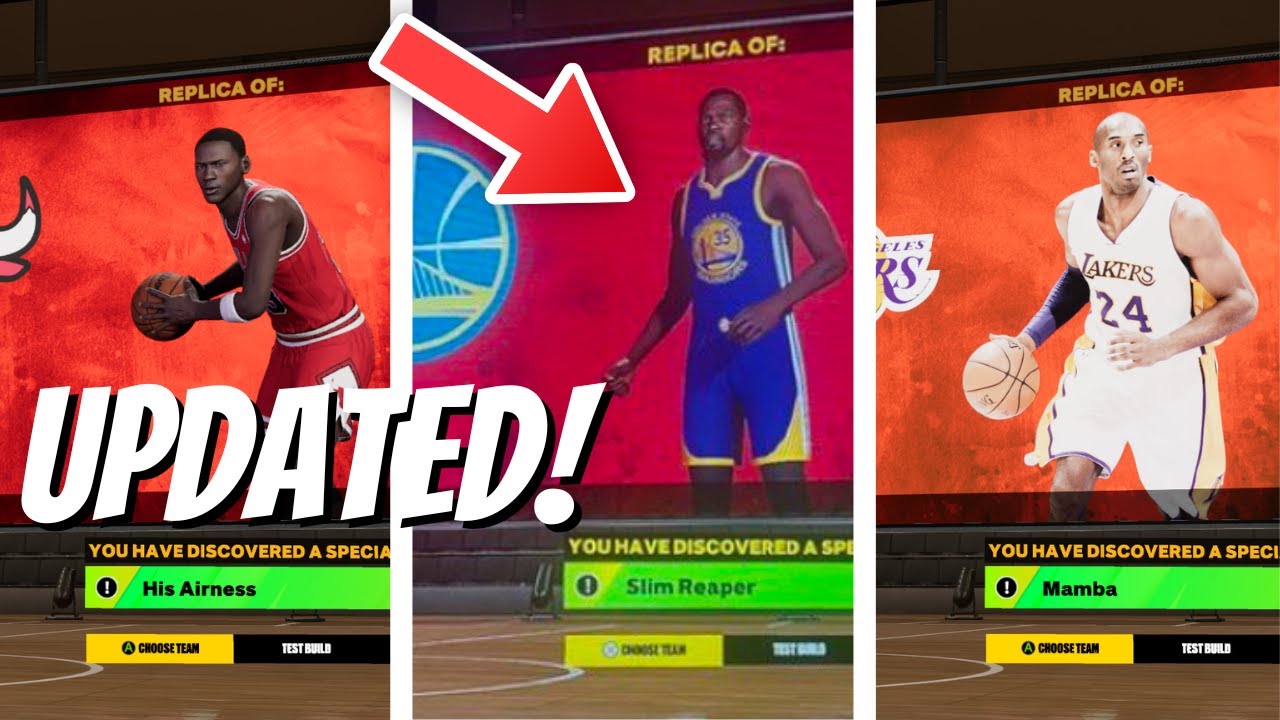The image consists of three horizontal rectangular screenshots side by side, each featuring different elements but maintaining a consistent layout. 

**Left Panel:**
- The bottom left corner prominently displays "Updated" in large white block letters.
- The screenshot itself shows a screen with the text "Replica of an Orange" at the top.
- Below this text, a basketball player is visible, wearing a red jersey and shorts.
- At the bottom, a yellow message states "You have discovered a SPECIA," but the sentence is cut off.
- Beneath this message, a lime green box features icons and text. On the left side of the box, there is a white eye symbol inside a black circle.
- To the right, in bolded black letters, it reads "His Airness," with "AIR" and "ESS" emphasized.
- Below this text, a yellow button labeled "Choose Team" is present next to a black button labeled "Test Build."

**Middle Panel:**
- Similar to the left panel, the text "Replica of an Orange" appears at the top.
- This panel features a basketball player in a blue jersey and shorts.
- A large red arrow, outlined in white, points downward at the player, labeled "Batman."
- At the bottom, the text in the lime green box reads "Slim Reaper," replacing the "His Airness" text from the left panel.
- The yellow "Choose Team" button and the black "Test Build" button are also present at the bottom.

**Right Panel:**
- This panel introduces another basketball player, this time wearing a white Lakers uniform.
- Once again, the top text reads "Replica of an Orange."
- In the lime green box at the bottom, the text "Mamba" replaces the previous labels from the other panels.
- Just like in the other panels, the yellow "Choose Team" button and black "Test Build" button are displayed at the bottom.

Each panel highlights different basketball players along with their respective nicknames, maintaining a cohesive aesthetic throughout the series of images.